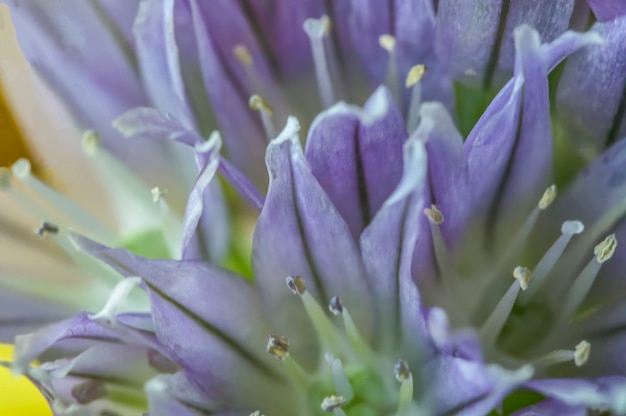This is an up-close, macro photograph of stunning purple-blue flowers, possibly a type of lily, with each bloom featuring six to eight pointed petals. The petals have pronounced black lines down their centers and range from light purple to darker shades. In the middle of the flowers, there are light green centers surrounded by white stamens with brownish nodules on the ends. The photo is tightly focused on the central flowers, with additional flowers slightly out of focus, creating a soft, blurred background. The bottom left corner features an indistinct yellow object, and more purple flowers extend to the upper right. The varying focus highlights the intricate details of the petals and stamens, emphasizing the natural beauty of the blossoms.